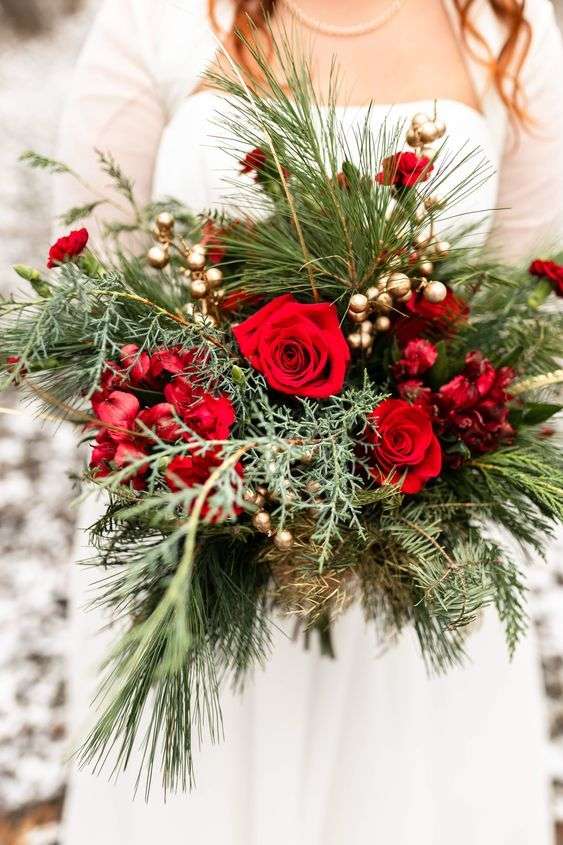This vertical, rectangular image prominently features a detailed wedding bouquet held by a woman. The bouquet is the focal point, with various elements arranged intricately. It comprises pine needles and pine tree vegetation as a base, adorned with vibrant red roses—one prominent rose in the center and additional roses at different positions within the arrangement. Surrounding the roses are smaller red flowers, possibly carnations, interspersed with clusters of gold-painted round objects, possibly artificial berries or decorative elements, as well as small silver balls.

In the background, partially obscured and out of focus, is the woman holding the bouquet. She is wearing a white wedding dress accompanied by a cream-colored, long-sleeved jacket that cuts off above her chest. Her auburn-to-brown tendrils of hair peep through the edges of the frame, below which a gold or pearl necklace is visible. The overall composition suggests a snowy backdrop, contributing to the seasonal and romantic atmosphere of the scene.